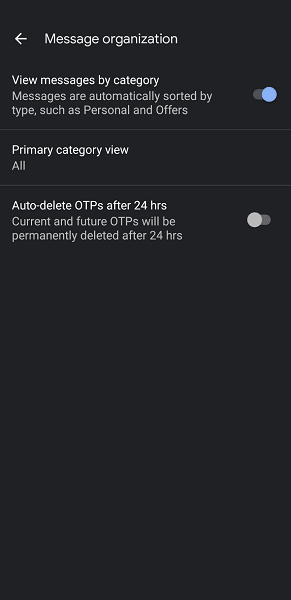The image features a sleek, user interface on a charcoal black background with white text providing detailed instructions and settings options. 

1. **Top Left Section**:
   - **Directional Arrow**: Positioned at the top left, pointing to the left.
   - **Text Label**: "Message Organization" is written next to the arrow.

2. **Main Body**:
   - **Section Label**: Beneath the directional arrow, the text "View messages by category" is displayed from left to right.
   - **Description**: Below, a line reads, "Messages are automatically sorted by type, such as Personal and Offers."
   - **Toggle Switch**: To the right of the description is a light blue toggle switch, labeled "Switch to On."

3. **Divider**: 
   - A light gray horizontal line spans from left to right beneath the above settings.

4. **Primary Category View**:
   - **Section Label**: The text "Primary Category View" is prominently displayed in white.
   - **Option**: The word "All" appears directly beneath.
   
5. **Divider**: 
   - Another light gray horizontal line runs from left to right, separating the sections.

6. **Auto-delete OTPs**:
   - **Feature Label**: "Auto-delete OTPs after 24 hours" is written in white text.
   - **Description**: Below this, the text reads, "Current and future OTPs will be permanently deleted after 24 hours."
   - **Toggle Switch**: To the right, another toggle switch in the shape of a small stretched oval is visible. This toggle is currently off, indicated by a light gray circle within a darker gray background.

The interface is visually organized with clear, distinct sections separated by light gray lines, and the toggles are designed with rounded edges for a modern, user-friendly appearance.